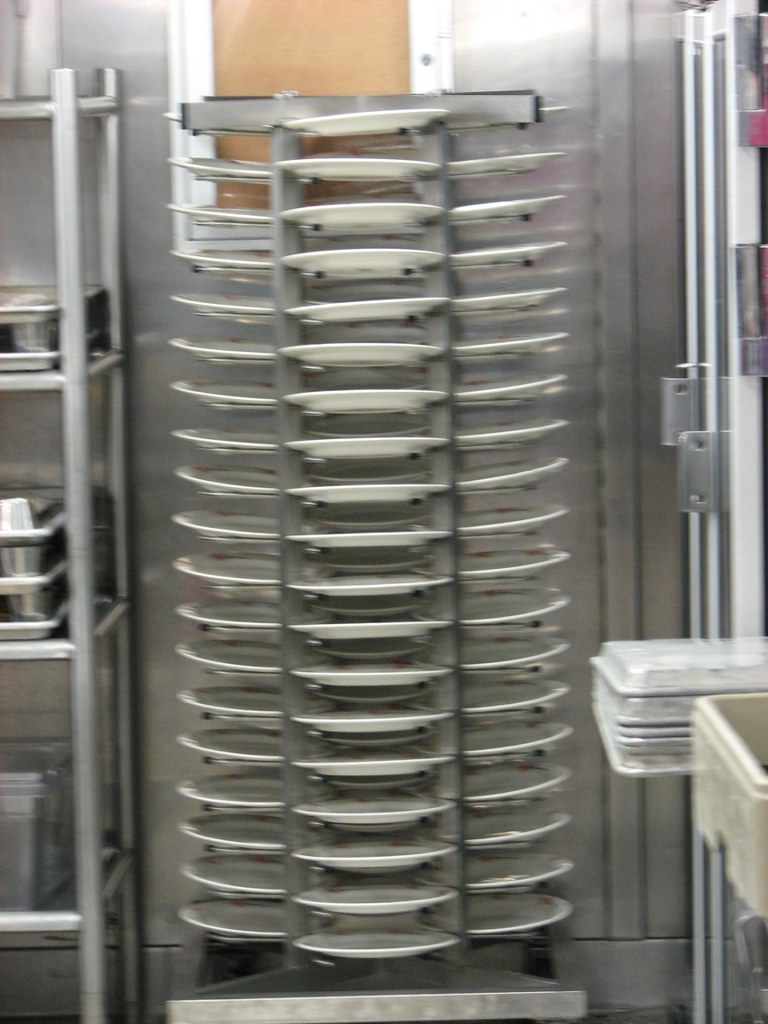This detailed color photograph, captured indoors in portrait mode, likely depicts an industrial or restaurant kitchen setting. The focal point is a tall, silver metal rack divided into three vertical sections, each section accommodating around 18 clean white dinner plates, stacked vertically with ample spacing. The rack is designed with small arms extending out to securely hold each plate in place. To the left of this rack, a partially visible silver case appears to store various baking pans or sheets, while to the right, multiple baking sheets are seen stacked upside down. The background reveals a silver wall with a white border and a brown corkboard-like detail, creating a visually organized and functional kitchen space. A tan basin, possibly for dishwashing, is also discernible towards the bottom right corner of the image.